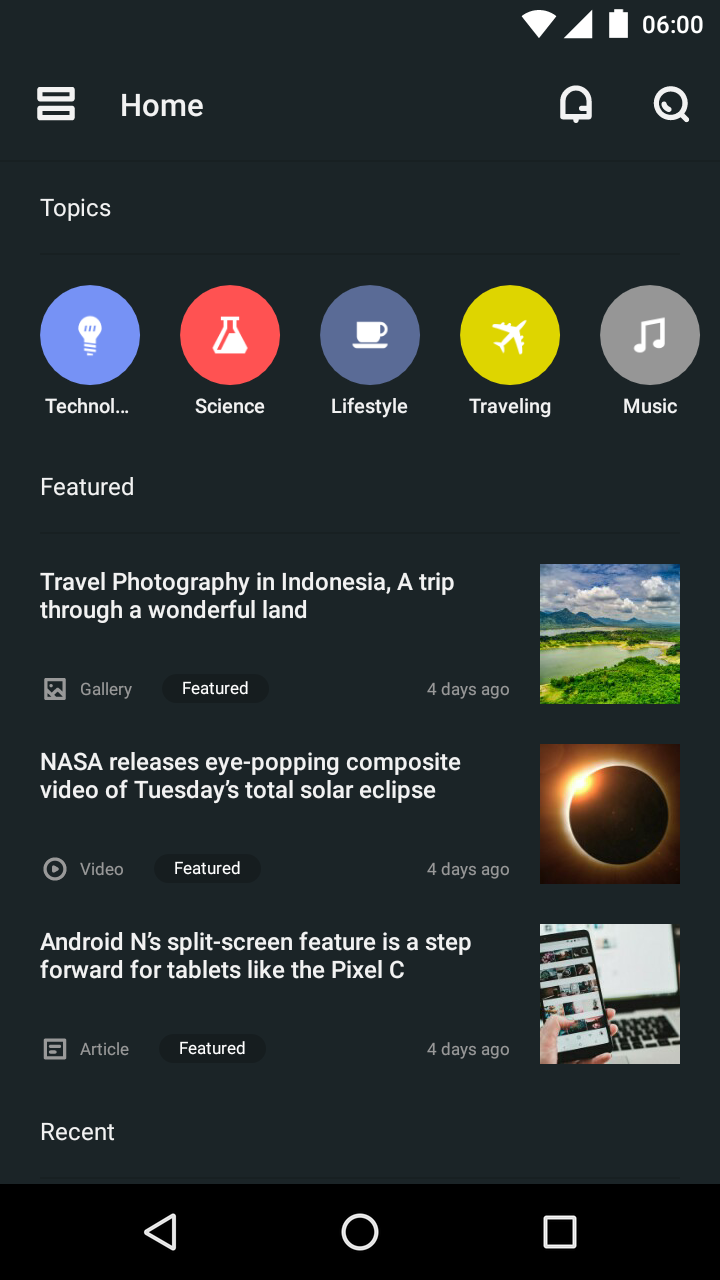The image appears to be a screenshot from a mobile phone displaying a dark gray background. At the top of the screen, the word "Home" is prominently featured, with "Topics" listed just below it. Underneath the "Topics" heading, there are five colored circles, each representing different categories:

1. The first circle is blue with a light bulb icon inside. It is labeled "Technologic" and says "Technolaw."
2. The second circle is red with a beaker icon, labeled "Science."
3. The third circle is a lighter gray with a coffee cup icon, labeled "Lifestyle."
4. The fourth circle is bright yellow with an airplane icon, labeled "Traveling."
5. The fifth circle is light gray with a musical note icon, labeled "Music."

Below these topic circles, the section titled "Featured" is visible. Under this section, there are two highlighted articles:

1. The first article is titled "Travel Photography in Indonesia: A Trip Through Wonderland" and is accompanied by a picturesque image. The image likely depicts Indonesia, featuring majestic mountains, a clear blue sky with clouds, a river, and lush green forests.
2. The second article discusses NASA's release of a stunning composite video of Tuesday's total solar eclipse.

The layout and vibrant icons make it easy for users to navigate and explore different topics.